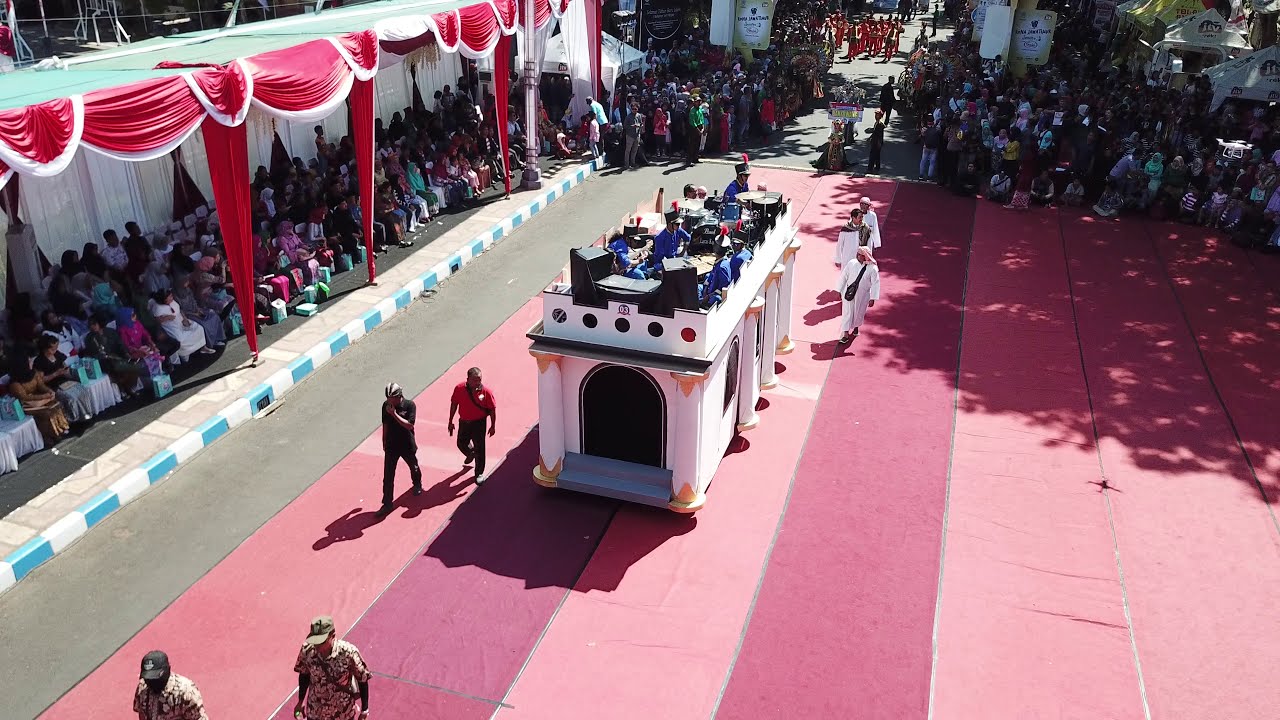In this photograph, we see a vibrant parade scene dominated by a central white rectangular float that appears to be inspired by Middle Eastern or Indian architecture. The structure features multiple columns and archways, with the main archway located at the bottom left, adorned with five distinct dots—gray, black, and red. On this float’s roof, a band performs, dressed in blue uniforms with black top hats adorned with a red feather. Various individuals surround the scene: to the left of the float, two people in black and red shirts walk, while two others dressed in camouflage, one wearing a black hat and the other a light green hat, are seen on the bottom left walking away. In the background to the right, three men dressed in traditional Middle Eastern white robes and red head wraps walk forward. The float and participants are positioned on an eye-catching ground made of vertical stripes—alternating light and dark pink—stretching across the ground and leading to a gray street bordered by a blue and white checkered curb. Above the street is a red canopy with white panels, and all along the fringes, diverse spectators dressed in various colors watch the procession, adding to the festive atmosphere. A large shadow, cast by the sun, also falls across the upper right corner of the scene.